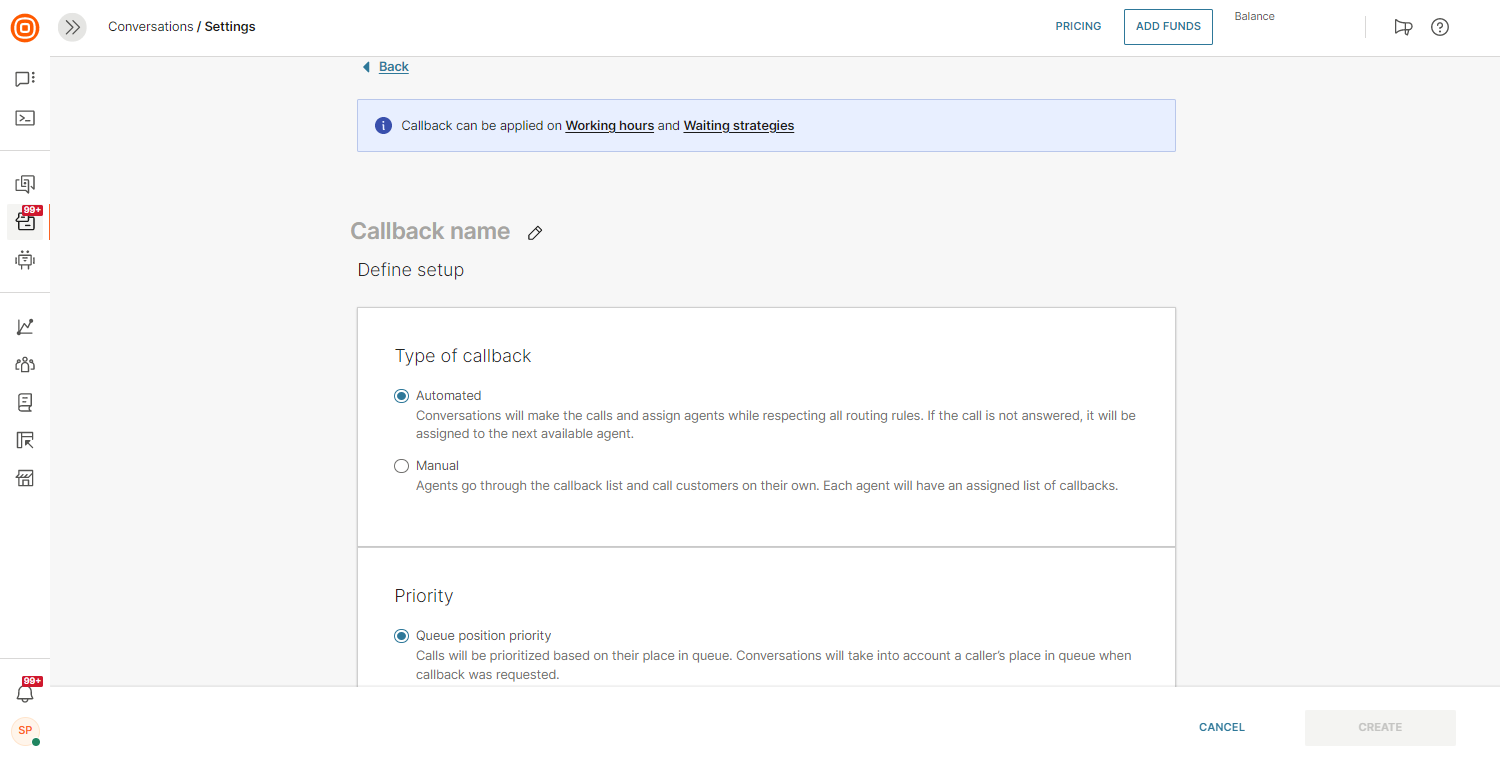### Detailed Caption

The image showcases a user interface for managing call-back settings with several detailed elements. At the very top, there is a tab labeled "Conversation Settings." Directly opposite this tab, on the right side, the word "Price" is displayed in blue text, next to which is an "Add Funds" button, enclosed in a blue box. To the right of this, there is a balance display, a loudspeaker emoji, and a question mark icon, likely indicating help or information.

On the far left side, adjacent to the "Conversation Settings" tab, is a double arrow pointing to the right, next to which is an orange circle with white squares around it, resembling a logo or a status indicator. Below this orange circle, there is a thin vertical column containing various icons: a comment bubble, a square with mathematical formulas, and a document icon labeled "99+" indicating numerous notifications or documents.

In the main document area, the top center features a "Back" button for navigation. Below this, there is a prominent blue box with the text "Callback can be applied on working hours and waiting strategies." This box highlights "working hours" and "waiting strategies" in bold black text to signify their importance. Below this, there are several lines of text followed by a section labeled "Callback Name," accompanied by an edit button and a pencil icon.

Under the "Callback Name," there is a field labeled "Define Setup" and a white input box. Further down, under the "Type of Callback" section, there are options for "Automated" or "Manual" callbacks with descriptive text explaining each option. The "Automated" option is currently selected, indicated by a blue dot. 

Lastly, the section for "Priority" features a blue dot and the text "Queue Position Priority." It explains that calls will be prioritized based on their position in the queue, taking into account the caller's place in the queue when the callback was requested.

This detailed interface likely belongs to a customer service or call center management system where precise configuration of callback settings is essential for operational efficiency.